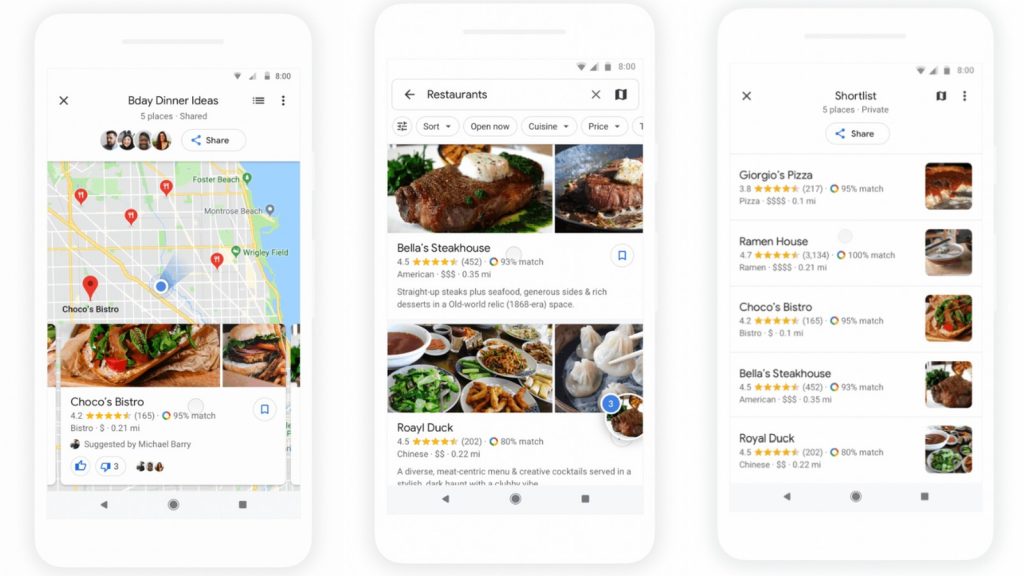**Caption:**

**Birthday Dinner Ideas: A Curated List of Top Five Spots**

Discover a selection of top-rated dining options perfect for a memorable birthday dinner, complete with photos, details, and a location map to help you choose the best place for your celebration. 

1. **Chacho's Bistro** - *Recommended by Michael Berry*
   - **Rating:** 4.2 stars
   - **Cuisine:** Sandwiches and casual fare
   - **Description:** A cozy bistro offering a variety of sandwiches, perfect for a laid-back dinner.

2. **Bella's Steakhouse**
   - **Rating:** 4.5 stars
   - **Cuisine:** Steakhouse
   - **Description:** Housed in an 1866-era space, Bella's Steakhouse features succulent steaks, seafood, generous sides, and rich desserts. The highlight is their steak topped with decadent herb butter, setting an old-world ambiance that’s perfect for special occasions.

3. **Royal Dock** 
   - **Rating:** 4.3 stars
   - **Cuisine:** Chinese
   - **Description:** Featuring a meat-centric menu and creative cocktails, Royal Dock offers an innovative take on Chinese cuisine in a stylish setting. 

4. **Joe’s Pizza**
   - **Rating:** 3.8 stars
   - **Cuisine:** Pizza
   - **Description:** Known for its classic and favorite pizzas, Joe’s Pizza is ideal for anyone wanting a more casual and fun dining experience.

5. **Ramen House**
   - **Rating:** 4.7 stars
   - **Cuisine:** Japanese
   - **Description:** Ramen House serves up hearty and flavorful ramen, making it a top choice for noodle lovers seeking an authentic Japanese meal.

Each restaurant on the list is marked on an accompanying map, ensuring you can easily locate and make reservations for your perfect birthday celebration spot.